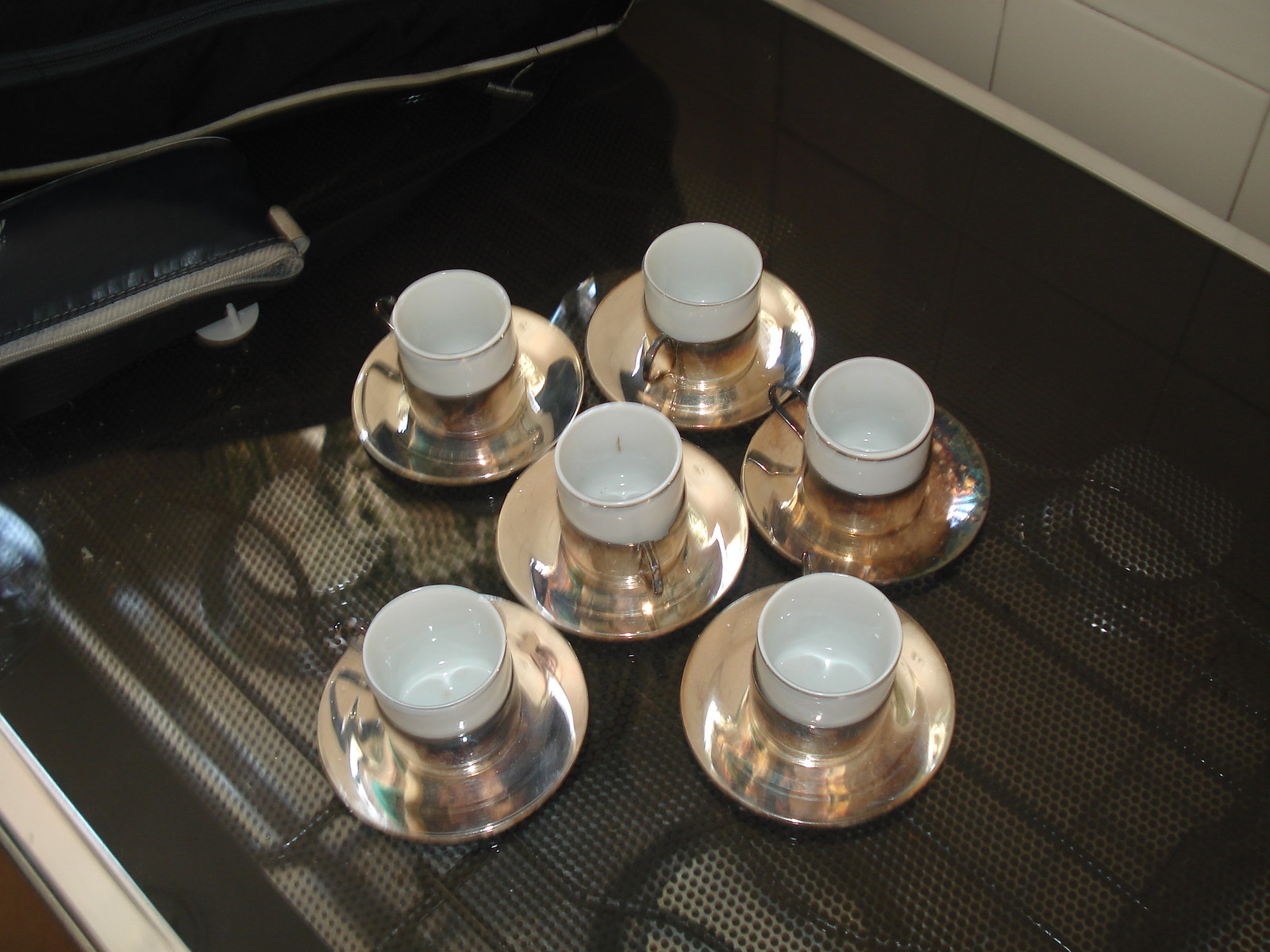The photograph showcases six elegant white teacups with delicate bronze rims, each nestled in matching bronze-colored saucers. The saucers feature slightly curved edges that create an area for the teacups, which also boast intricate handles exhibiting a mix of bronze and a hint of silver. These teacups and saucers are meticulously arranged on a gas stove burner, its black grate revealing the silver burners beneath. The light in the room captures reflections on the bronze surfaces, further enhancing the sophisticated design. The cups appear to be meant for a strong tea, possibly Turkish, with each cup capable of holding about half a cup of liquid. The setting suggests a ceremonial aspect, possibly involving a samovar for serving. Additionally, to the right part of the image, there's a notable presence of two black bags with cream-colored zippers, adding an extra layer of context to the scene.